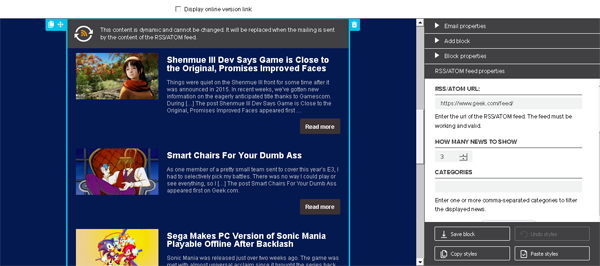This image features a dark blue background on the left side and a black banner across the top with a white, hard-to-read text that seems to state: "This content is dynamic and cannot be changed. It will be replaced when the feed is sent. Try the content of the feed." Below the banner are three thumbnail images of cartoons, each accompanied by white text labels. The first thumbnail is labeled "Shin Miu 3," with a subheading that reads, "Dev says game is close to the original, promises improved faces," followed by a paragraph of text and a "Read More" button. The second thumbnail is titled "Smart Chairs for Your Dumb Ass," also followed by a paragraph of text and a "Read More" button. The third thumbnail reads, "Sega makes PC version of Sonic Mania playable offline after backlash," with similar accompanying text and a "Read More" button.

On the right side of the image, there is an area containing a series of dropdown menus in black with white text. These menus are labeled as follows: "Email Properties," "Ad Block," "Block Properties," "RSS Feed Properties," "URL," with a prompt to "Enter the URL," and "Feed" with a note that "The feed must be working and valid." Additionally, there is an option for "How many news to show," and a section for "Categories," which is left blank.